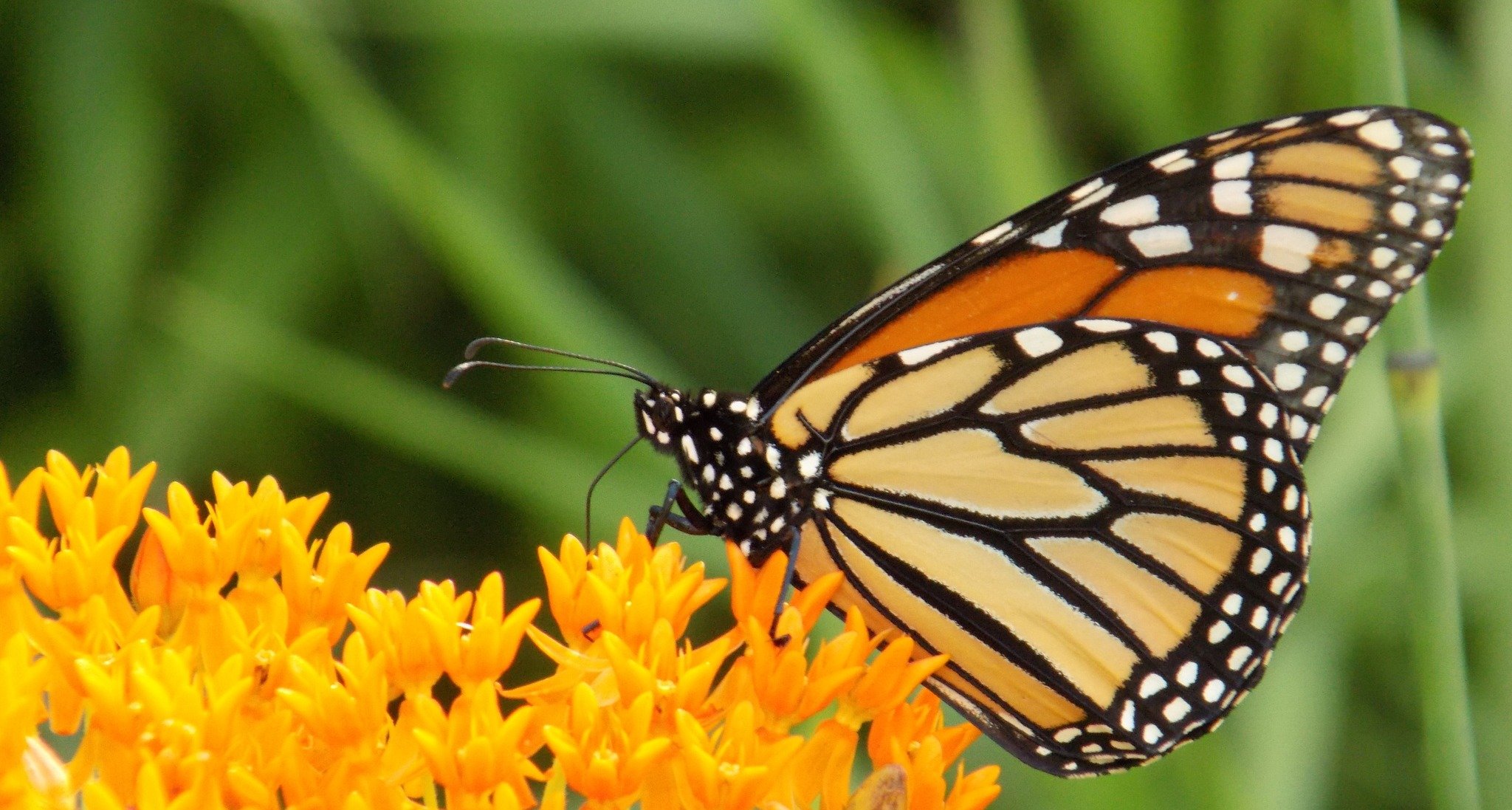In the photograph, a captivating monarch butterfly is perched delicately atop a cluster of vivid, yellow lantana flowers situated in the lower left corner of the image. The butterfly, prominently displayed in the foreground, boasts striking wings adorned with a blend of orange, yellow, brown, and white patterns, while its black wings are edged with white spots. The details are so fine that one can clearly see the butterfly's antennae and its proboscis extending into one of the flowers, sipping nectar. The butterfly's body also features distinct white spots. The vibrant colors of the butterfly and flowers stand out sharply against the blurred background, which consists of various shades of green foliage, including tall grass or reeds, adding a gentle, natural ambiance to the scene. The detailed close-up allows even the individual legs of the butterfly to be visible, enhancing the intricate beauty of this moment in nature.